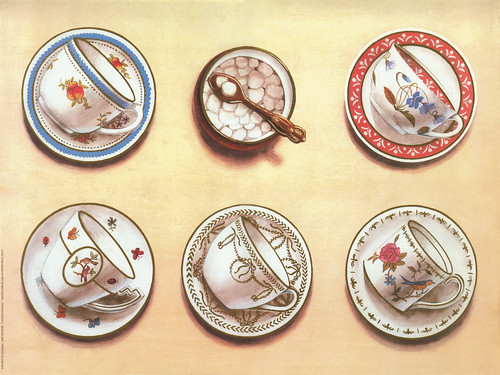The image depicts a detailed and colorful painting featuring five coffee mugs, each lying on its side on matching saucers, all set against an off-white background, possibly a table or tablecloth. Each cup and saucer set exhibits intricate designs:

1. **Top Left:** A white cup and saucer with a blue border. The cup features a yellow flower with green leaves, matching the floral pattern on the saucer.
2. **Upper Right:** A white cup and saucer with a red border. The saucer has white details within the red border, and the cup displays blue flowers with curly stems and green leaves.
3. **Bottom Left:** A white cup and saucer set adorned with orange and blue flowers and painted butterflies. The cup has an oval design in the middle featuring two birds and an orange butterfly with a leaf.
4. **Bottom Middle:** A white cup and saucer designed with green patterns. The saucer has a laurel wreath with red bows, matching the green scalloped edges on both the cup and saucer.
5. **Bottom Right:** A white cup and saucer set with green-like leaves along the borders. The cup features a red rose with green leaves and a twig with a blue and yellow bird.

Additionally, on the left side among the cups is a sugar bowl filled with sugar cubes, accompanied by a brownish-gold spoon holding a couple of sugar cubes. The meticulous detailing and arrangement of the cups and saucers highlight the careful craftsmanship and aesthetic appeal of the artwork.